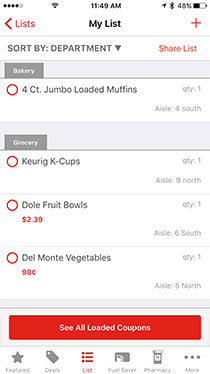The image depicts a mobile application interface focused on grocery shopping. At the top, there is a heading labeled "My List," which displays various food items. The first item is "Four Count Jumbo-Loaded Muffins," listed under the bakery section. The grocery section includes items such as Keurig K-Cups, Dole fruit bowls, and Del Monte vegetables, each with a notation indicating a quantity of one.

At the bottom of the list, a button labeled "CL Loaded Coupons" suggests the availability of digital coupons for the listed products. A "Sort By" option allows users to organize items by department or food type. Additionally, there is a share button for easy sharing of the list.

At the very bottom of the screen, there are several subsections: Featured Deals, List, Fuel Saver, and Pharmacy. The active selection is "List." The presence of a "Fuel Saver" section implies potential fuel discount offers, possibly indicating a partnership with stores that also have pharmacies, such as CVS or Walgreens.